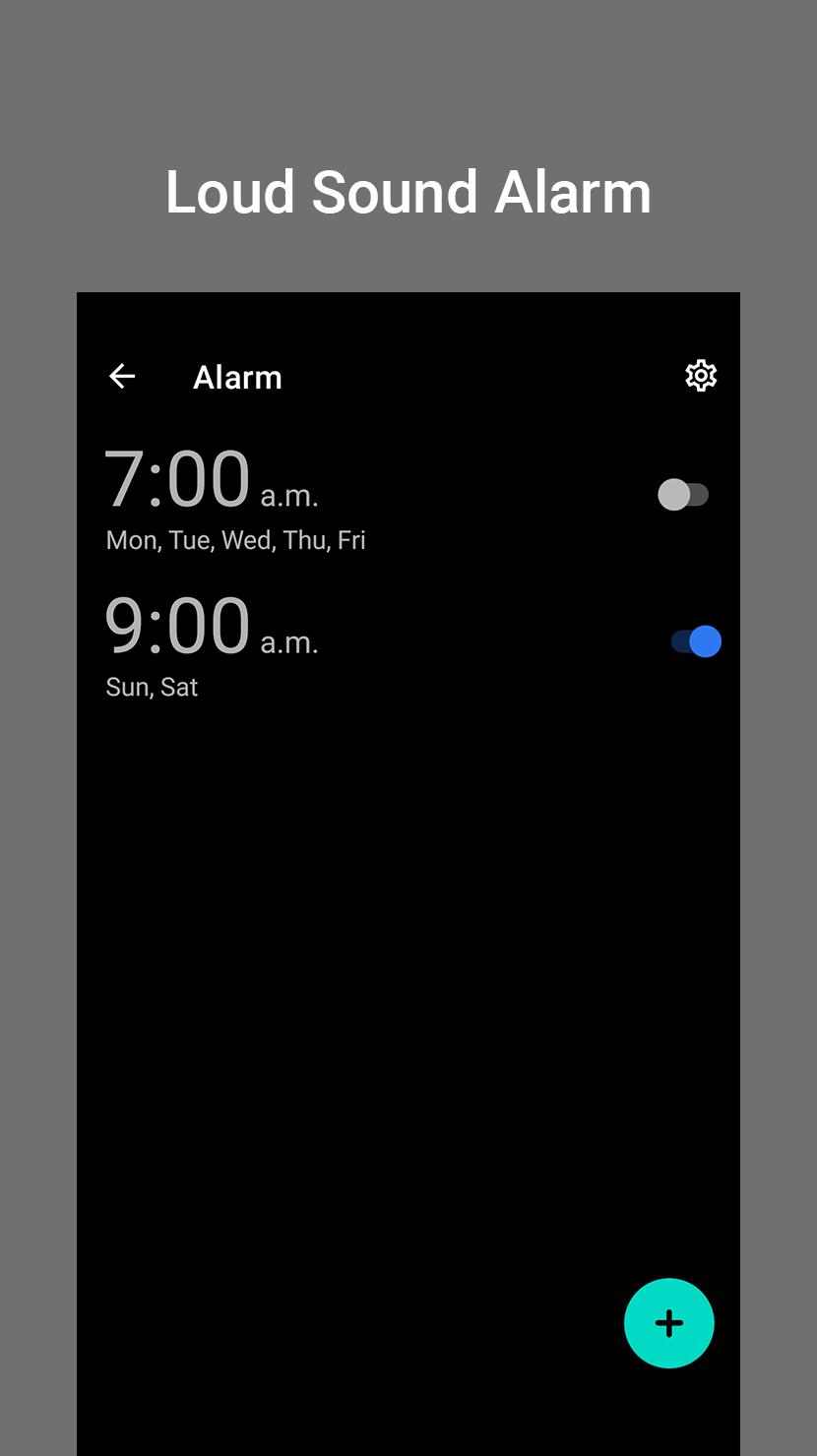The edited screenshot displays an iPhone alarm settings screen with a black background, showcasing a cropped view. On the top left, bold white text reads “Alarm,” accompanied by a left-pointing arrow for returning to the clock settings. On the top right, a cogwheel icon indicates settings options. Below, a vertical list of alarms appears: the first alarm, shown in large grey letters, is set for 7:00 AM and specifies the weekdays (Monday through Friday), with its toggle switch turned off. The second alarm, set for 9:00 AM, includes the weekend days (Saturday and Sunday), with its toggle switch turned on. At the bottom center, there is a blue circle containing a black plus icon, intended for adding a new alarm. The overall background transitions to grey, and the alert text at the top reads “Loud Sound Alarm.” The screenshot is angled slightly towards the bottom of the grey section, emphasizing the listed alarms and their settings.